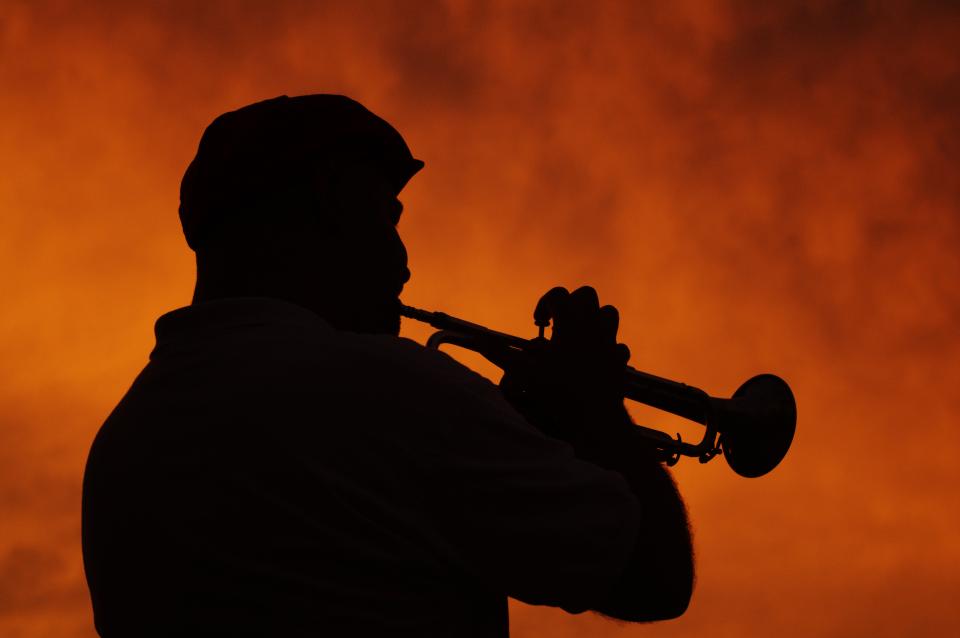This evocative photograph captures a solemn, silhouetted portrait of a trumpet player against a dramatic, smoky burnt orange sky with dark reddish-black clouds, fading to a deep brown at the edges in a vignette style. The musician's thick torso emerges from the bottom left, leading to his right arm which angles downward before curling back up, where his four fingers delicately rest on the trumpet's keys. His head, tilted downward in a somber pose, displays rounded cheeks, the outline of a prominent nose, a sharp brow, and the distinct silhouette of a flat cap. Enhanced by a little light behind one sleeve, the texture suggests he is donned in a fluffy sweater or collared jacket. The trumpet, slightly angled downward to the right, features a dark tube on top and an oval exit at the end. The overall image conveys a reflective, melancholic atmosphere, likened to a soldier playing a poignant tune such as taps.